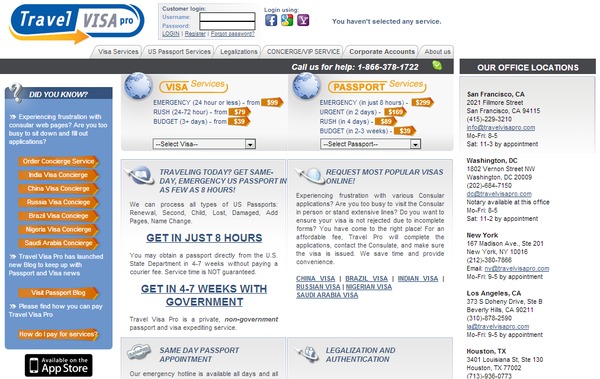The webpage for Travel Visa Pro is bustling with information and functional elements aimed at facilitating travel documentation services. At the top, the Travel Visa Pro logo features prominently: the word "Travel" in white text set against a blue and white oval background, and "Visa" in gray with "Pro" in a shade of blue. A yellow arrow curves around the bottom of this oval, pointing right.

Directly below the logo is a customer login section where users can enter their username and password, with links for "forgot password" and "register." There's also the option to log in using Facebook, Google, or Yahoo, each represented by their respective icons.

The webpage indicates that no service has been selected yet and showcases a horizontal navigation bar with tabs for Visa Services, U.S. Passport Services, Legalizations, Concierge/VIP Service, Corporate Accounts (highlighted), and About Us.

A prominent gray bar offers help with a call-to-action: "Call Us for Help," listing two potential phone numbers, 1-866-XXX-XXXX and 1-855-378-1722. There's also a "Did You Know" section, alongside another critical segment detailing emergency services offering U.S. passports in as fast as eight hours.

Below this, users can find more information about popular visas and urgent passport services, followed by various blurbs. On the left side, an array of nine large orange arrows directs users to specific services such as India Visa Concierge, China Visa Concierge, Russian Visa Concierge, and so forth.

On the right side, there's a comprehensive list of Travel Visa Pro's physical locations in San Francisco, Washington, D.C., New York, Los Angeles, and Texas, supported by an icon indicating the availability of a mobile app on the App Store, highlighted by an image of a smartphone.

This detailed, multi-faceted layout ensures users have easy access to all the necessary tools and information to manage their travel documentation efficiently and effectively.